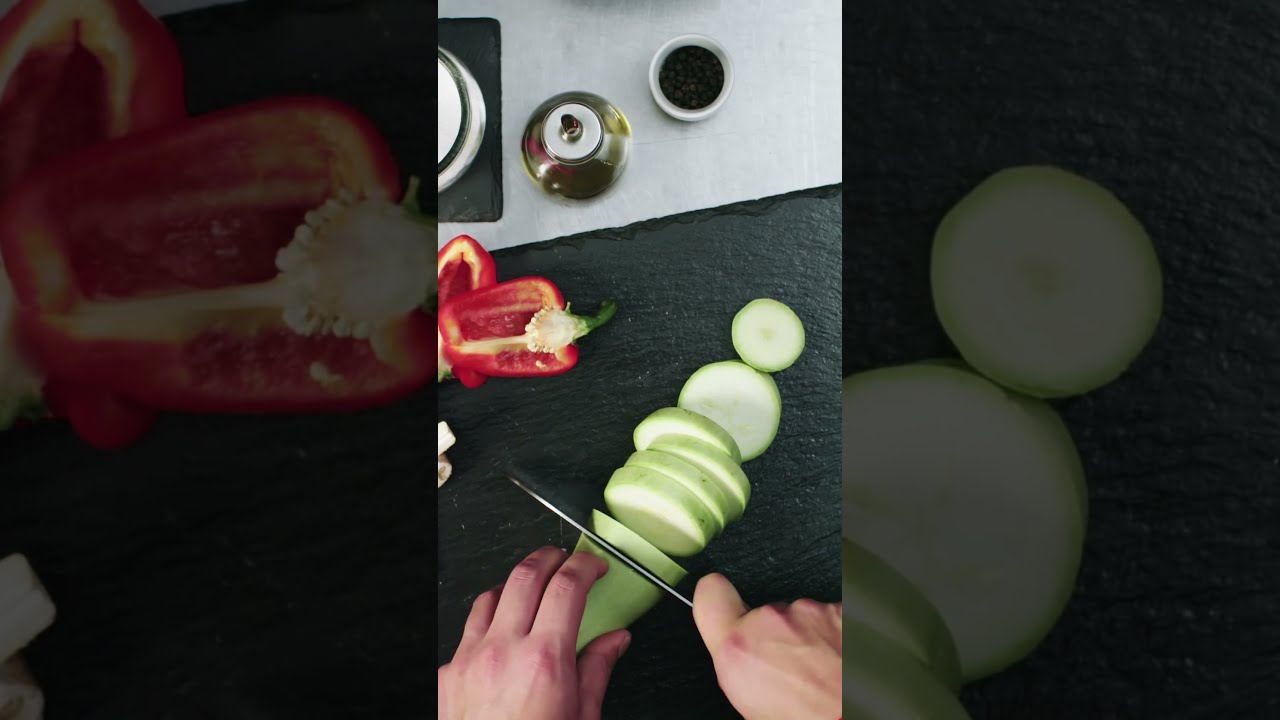The image depicts a detailed culinary scene on a black cutting surface. There are two human hands with light-colored skin in the bottom portion of the image. The right hand is skillfully using a knife to slice a pale green zucchini, with the vegetable being cut into even slices. To the left, there is a halved red pepper, revealing its seeds. The black cutting surface transitions into a white surface at the top of the image. Positioned on this white surface is a golden tea kettle, flanked by a couple of white containers. On the right side of the kettle, there's a white cup filled with a dark liquid. On the left, a small, circular white container with a black-edged lid sits on a black patch. The scene is rich in colors, featuring green vegetables, red pepper, gold kettle, black and white surfaces, and various shades of skin tones, evoking the feeling of an intimate cooking session.